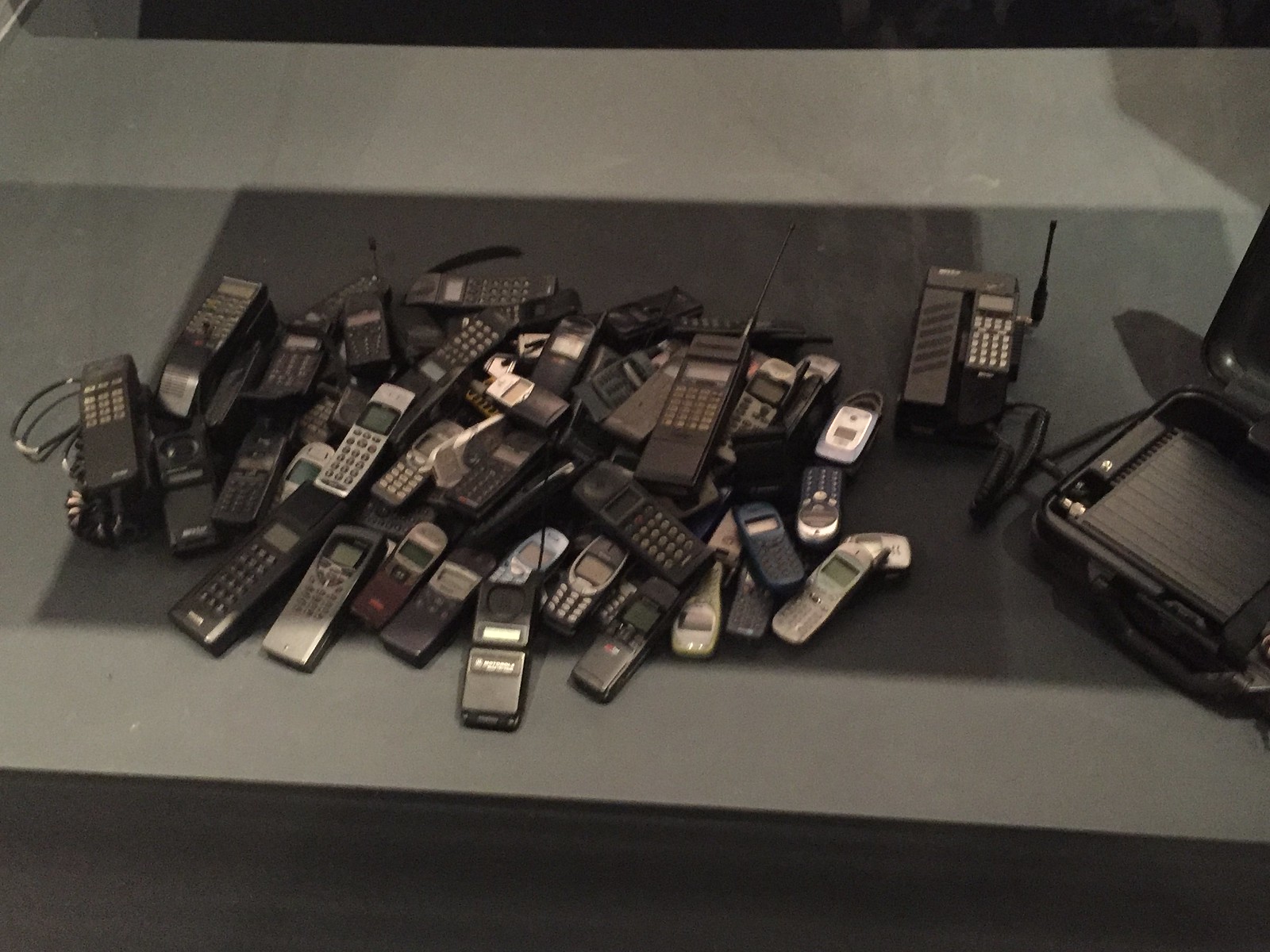This photograph, taken from a bird's eye view, captures a collection of approximately 30 vintage cell phones laid out on a multi-toned gray desk. The central focal point of the image is a large black rectangular area filled with these phones, ranging from small rectangular models to larger phones with antennas. Among the assortment, some phones even have long cords attached to them, indicative of older technology. The color palette of the phones spans shades of gray, black, and even hints of red, blue, and other monochromatic tones. Several of these phones are identifiable as flip phones, while others display the traditional compact design with small, non-color screens and button keypads characteristic of early cell phones like old Nokia models. On the right-hand side of the image, there is an open black case with a handle at the front, containing flat material inside, likely connected to one of the phones. The overall ambiance of the photograph is dimly lit, enhancing the nostalgic feel of this collection of obsolete mobile devices.